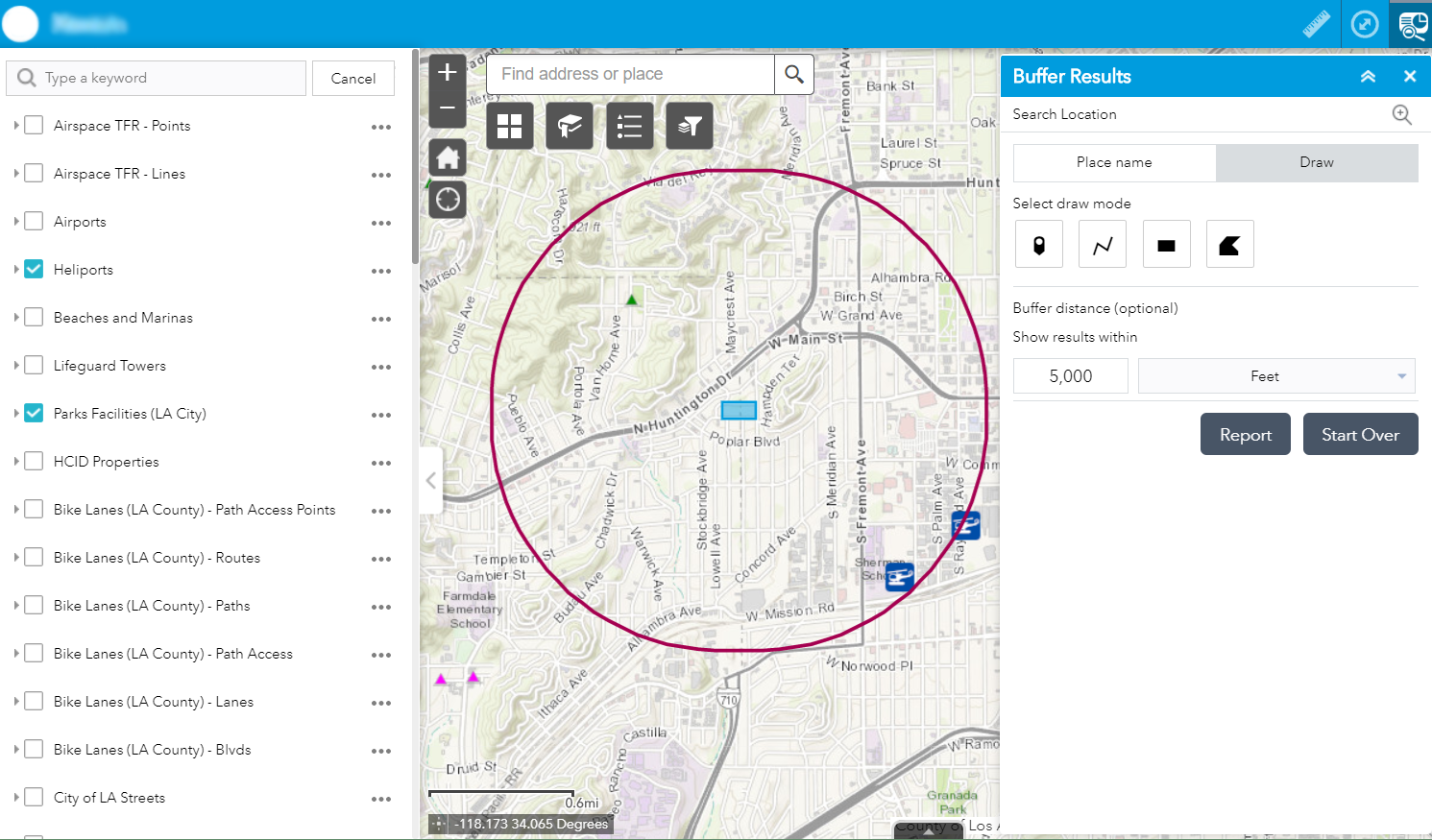The screenshot depicts a detailed interface of a website, divided into three sections: left, middle, and right. At the top of the page, a rich, lighter blue border spans across, with a white circle in the top-left corner containing a blurred-out name. On the right side of this border, there are three icons.

In the right section, beneath the blue border, there's a blue bar, and to the left within this bar, "Buffer Results" is displayed. Proceeding downwards, the background turns white. There's a search bar labeled "Search Location." Below this search bar, a white tab with black lettering reads "Place Name." Adjacent to this, a gray tab labeled "Draw Bar" in black text is visible. Further down, options for "Select Draw Mode" appear, featuring four squares with different emblems. Underneath, it reads "Buffer Distance Optional," followed by the text "Show Results Within" alongside a square labeled "5,000" and another labeled "Feet." Towards the bottom, two dark gray tabs with white lettering are present; the left tab reads "Report," and the right tab reads "Start Over."

The center section prominently features a map with a large dark red circle around its center. In the middle of this circle, a blue rectangle labeled "Poplar Boulevard" is displayed. The map primarily uses gray with a small amount of green in the upper-left corner and includes road names. At the top, a search bar reads "Find Address or Place." Below this search bar are four gray squares featuring icons. To the left, a vertical gray rectangle contains a white plus sign at the top and a white minus sign at the bottom. Additionally, there is a gray square with a home icon and a gray circle with a location icon inside.

In the right section, a search bar labeled "Type a Keyword" sits at the top, with the word "Cancel" in black to its right. Below are a series of squares, each paired with the names of airports or roads. The fourth and seventh squares down are blue with white checks, while the remaining squares are white. Corresponding names are listed next to each square, and on the far right side of this section, three ellipses are visible.